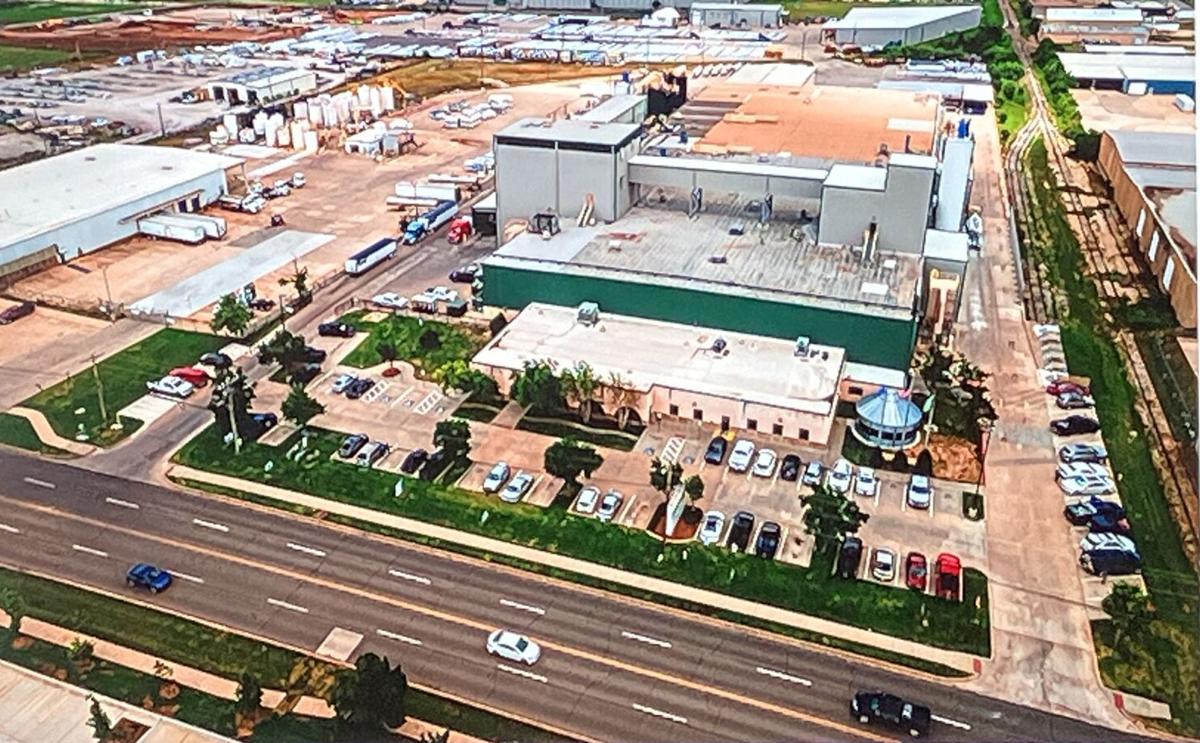This is a detailed aerial view of an industrial complex in an American city, captured during the daytime. At the bottom of the horizontally aligned, rectangular photo, there is a four-lane highway with a dashed white line divider, featuring a white car, a blue car, and a black truck. Across the highway, in the foreground, multiple parking lots are filled with approximately 20 to 30 cars. The central area of the image showcases a white single-level building, appearing as a corporate site, and directly behind it, a green building that resembles a manufacturing plant. Surrounding these key structures are additional parking lots, grass, trees, and several rectangular and stone or brick buildings, suggesting a bustling industrial worksite. On the left side of the photo, more industrial buildings and warehouses can be observed, indicating a well-developed industrial zone. In the upper left background, further parking lots and rectangular buildings are visible, reinforcing the area's industrial nature. The scene also includes some dirt portions and railroad tracks adjacent to the main building, enhancing the depiction of a dense and active industrial environment.